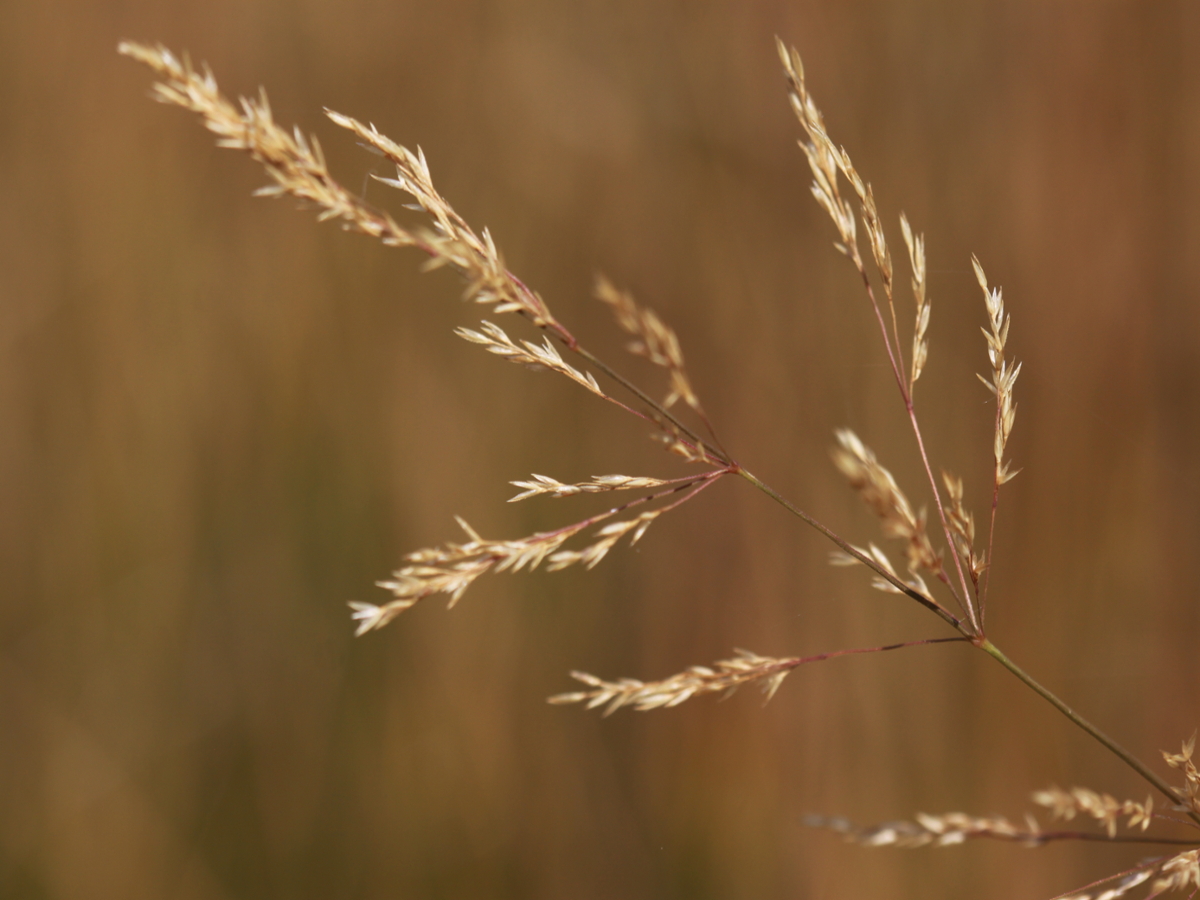This professionally shot photograph captures a delicate, grainy plant, reminiscent of wheat or hay, against a completely blurred, brown background. The image employs a shallow depth of field, highlighting the intricate details of the plant while rendering the background into an indistinct brown patch. Central to the composition is a thin, fragile green stem branching out into several smaller stems, each tipped with light brown, spike-like grains clustered in bundles. These fine, spiky structures and their tan hues blend subtly with the background, emphasizing the plant's texture and fragility. The image's diagonal composition accentuates the plant’s structure, creating an aesthetically pleasing and detailed visual experience.